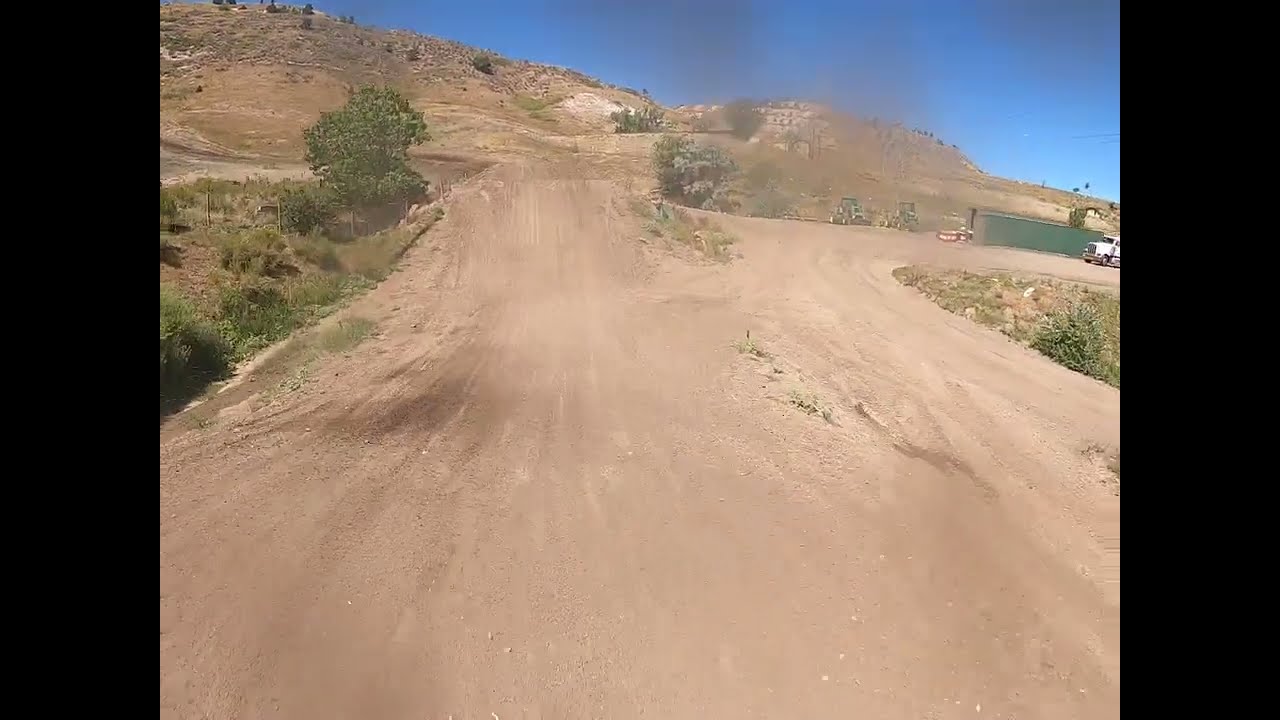The photograph captures an outdoor scene featuring a winding dirt path that might be a dirt trail or even a dirt bike ramp, set against the backdrop of a rugged mountain or tall hill. The terrain is marked by a mixture of dry, brown dirt interspersed with patches of grass, weeds, small shrubs, and a few trees, giving it a somewhat sparse and arid appearance, suggestive of either a desert or mountainous area. 

To the right of the dirt path, there is an area with a white tractor trailer and green storage containers approximately 20 feet long. Nearby, green outdoor tractor equipment is visible, along with a field that is rocky and slopes gently. In the background, you can see multiple building structures, contributing to a somewhat industrial or utilitarian feel to the scene. 

The sky above is a clear and vibrant blue, indicating that the image was taken during the daytime. Overall, the setting looks somewhat deserted and devoid of people or animals, highlighting its isolated and tranquil nature. 

The central dirt road seems to lead into a dirt parking lot or open area, emphasizing its utilitarian purpose. Both the road and the surrounding scenery underline the rugged and expansive character of this outdoor location.